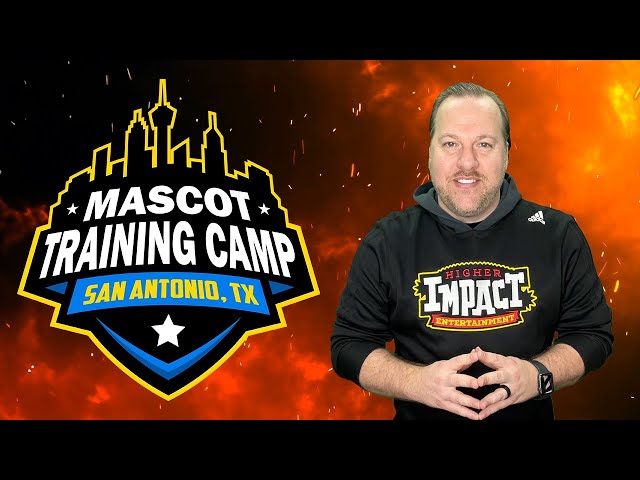In the image, a middle-aged Caucasian man stands on the right side, wearing a black hoodie with the words "HIRE IMPACT ENTERTAINMENT" prominently displayed on the front. The text appears in a combination of red, white, and yellow, with "HIRE" in red letters, "IMPACT" in large white letters, and "ENTERTAINMENT" in yellow letters on a red banner beneath. The man has short, combed-back brown hair, a stubble beard, and a high forehead. His hands are pressed together in front of him, displaying a black ring on his left hand and a smartwatch on his wrist. 

The backdrop behind him features dramatic orange and black hues reminiscent of fire or an explosion. To the left of the man is a logo with an outlined image of the San Antonio skyline atop a black background with a yellow border. The logo contains white text reading "MASCOT TRAINING CAMP." Below this are the words "SAN ANTONIO, TEXAS" in yellow on a blue banner. This image serves as an advertisement for a mascot training camp in San Antonio, Texas.